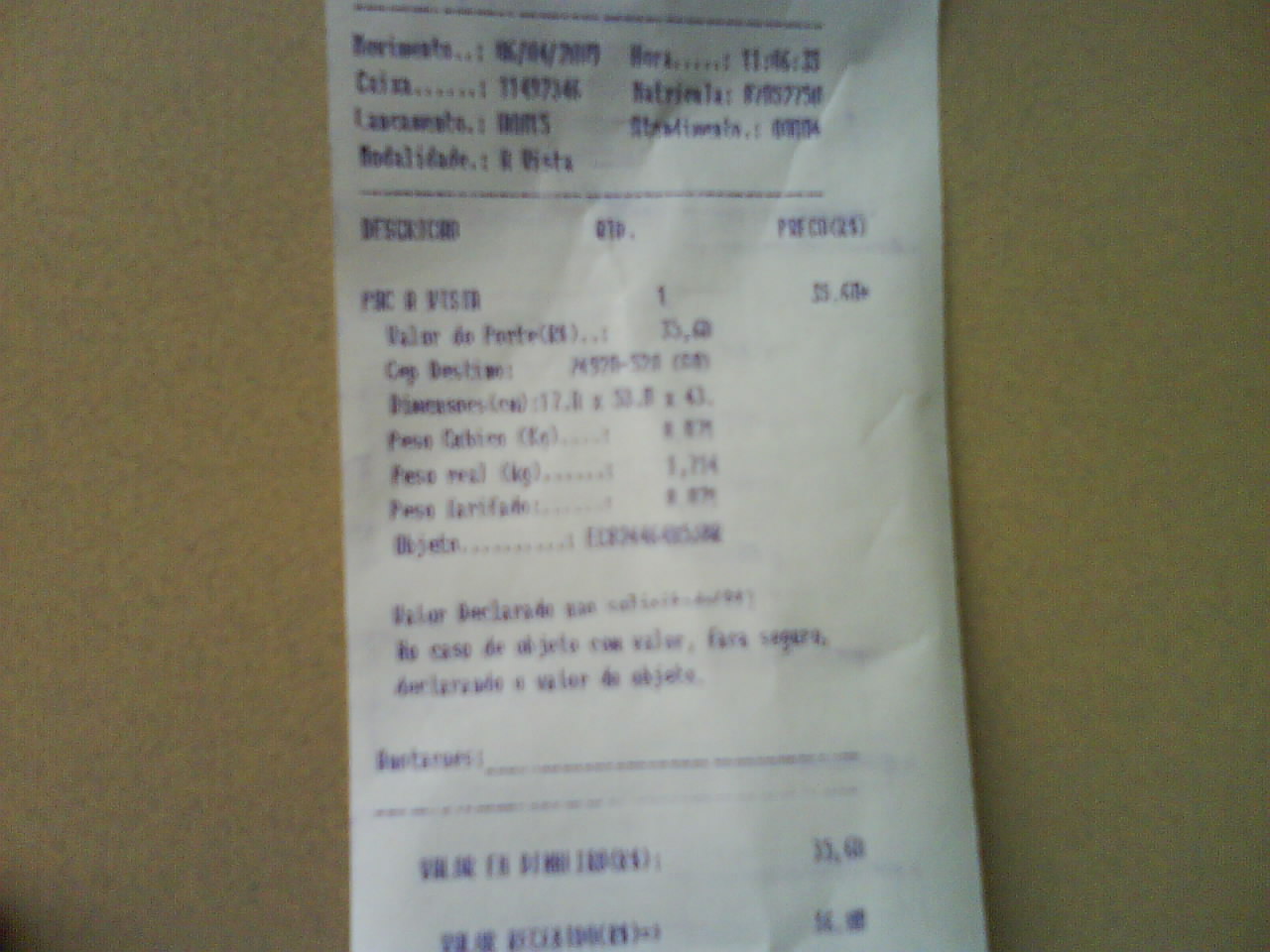This is a photograph of a white, rectangular receipt showcasing blue-colored text. The receipt, listing multiple purchased items, appears to be either written in a non-English language or is too blurry to decipher clearly. The total amount spent is visible as $35.60. The receipt rests on a light brown surface that could be cardboard. Additionally, the receipt shows signs of being wrinkled, suggesting it may have been crumpled previously. Toward the top of the receipt, there is likely information detailing the date and time of the transaction. At the bottom, one can see the order total alongside possible tax or tip details.